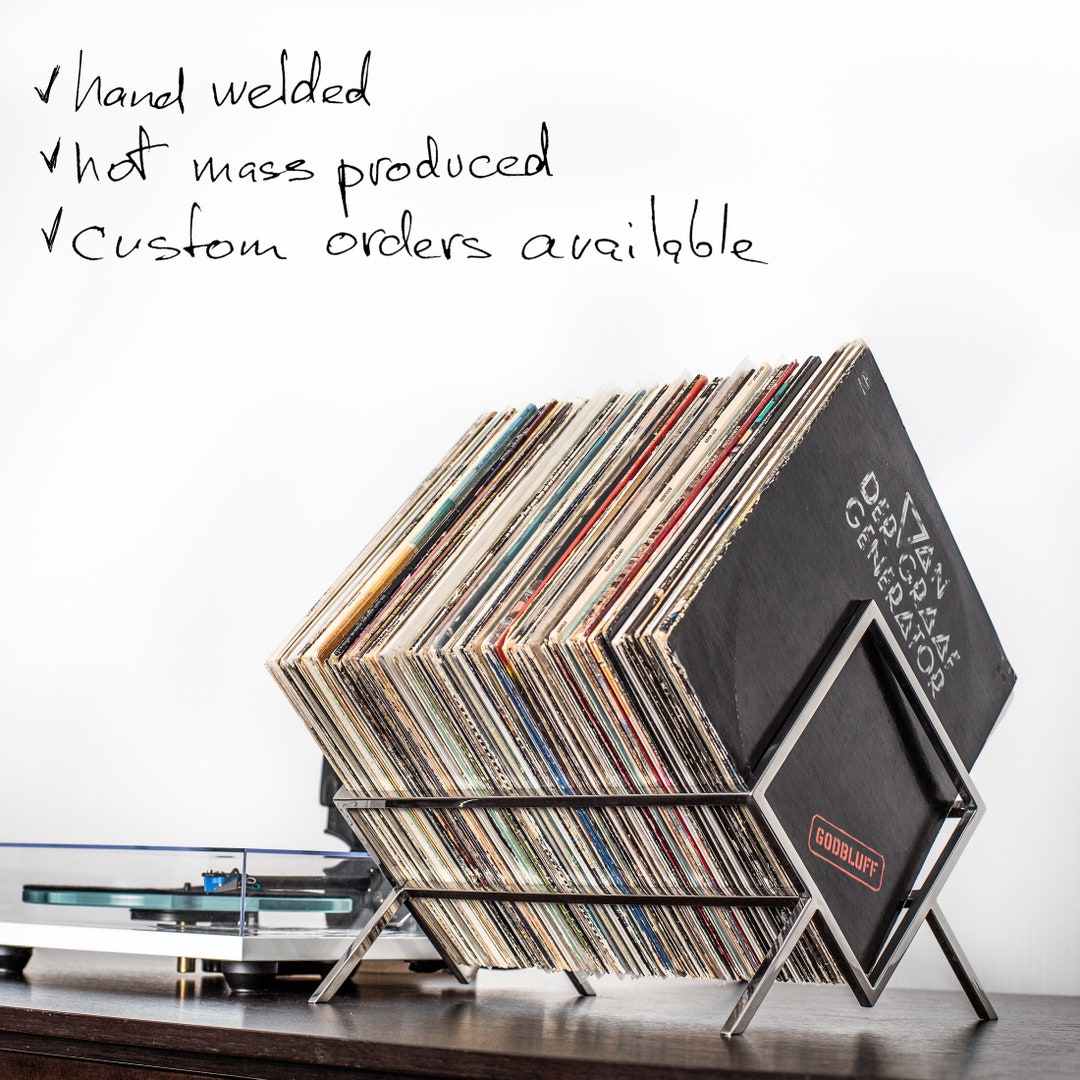The photograph, taken indoors, captures a vertically rectangular scene against a light gray, almost white, wall. A wooden table with a dark brown surface spans the bottom of the image. On the left side of the table sits a turntable with a white base and black legs, featuring a teal interior and a clear plastic cover adorned with a light blue line across it. Handwritten text in the upper left corner lists three attributes, each marked with a checkmark: "Hand Welded," "Hot Mass Produced," and "Custom Orders Available."

To the right of the turntable, a sleek, silver metal stand holds a collection of records. The stand has a unique design, with two metal pieces extending from the right to the left to support the records from the bottom. The foremost record on the right is black, displaying a label in the bottom right corner that reads "Coles Bluff" in red, encased in a line. The top part of the label is branded with the name "DED ZAN Generator." The background is an unobtrusive light gray, emphasizing the featured items on the wooden table.